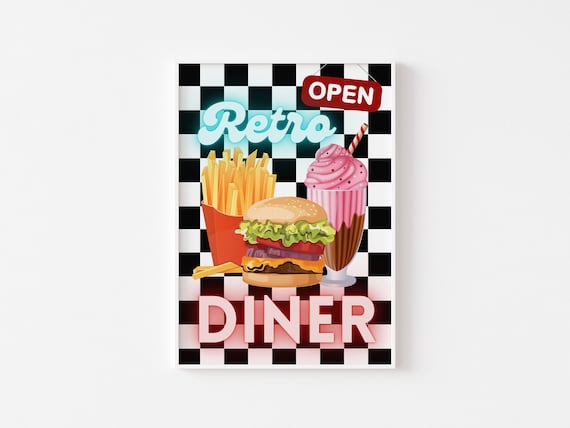A vibrant poster for a retro diner featuring a clean white background with a black and white checkered pattern. At the top right, a red tag with "Open" in white text sets a welcoming tone. Centrally, a striking image of a classic hamburger garnished with lettuce, tomato, onion, and an orange-brown meat patty. Surrounding the burger, a strawberry milkshake with a candy-cane striped straw, and a serving of fries in a red container capture the essence of classic diner fare. The words "retro diner" appear in bold neon blue and red lettering, invoking a nostalgic atmosphere. The entire design is clean and visually appealing, effectively capturing the retro diner theme.